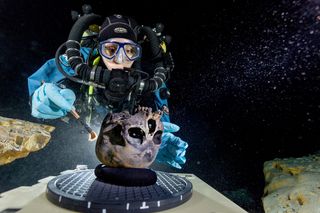The image depicts a scuba diver in a predominantly blue wetsuit with matching goggles and gloves, complemented by black scuba gear including a breathing apparatus and helmet. The diver is examining a peculiar round, brownish object with multiple holes, which bears some resemblance to an alien entity or an unusual underwater specimen. The object is positioned on a large, man-made mat-like structure. The composition of the scene includes some surrounding rocks and a few yellow and white accents, creating a contrast against the predominantly dark, almost black background that suggests deep underwater exploration. The diver appears to be carefully inspecting or brushing the object, possibly as part of an archaeological or scientific study. The presence of bubbles confirms the underwater setting, and there are no textual elements present in the image.